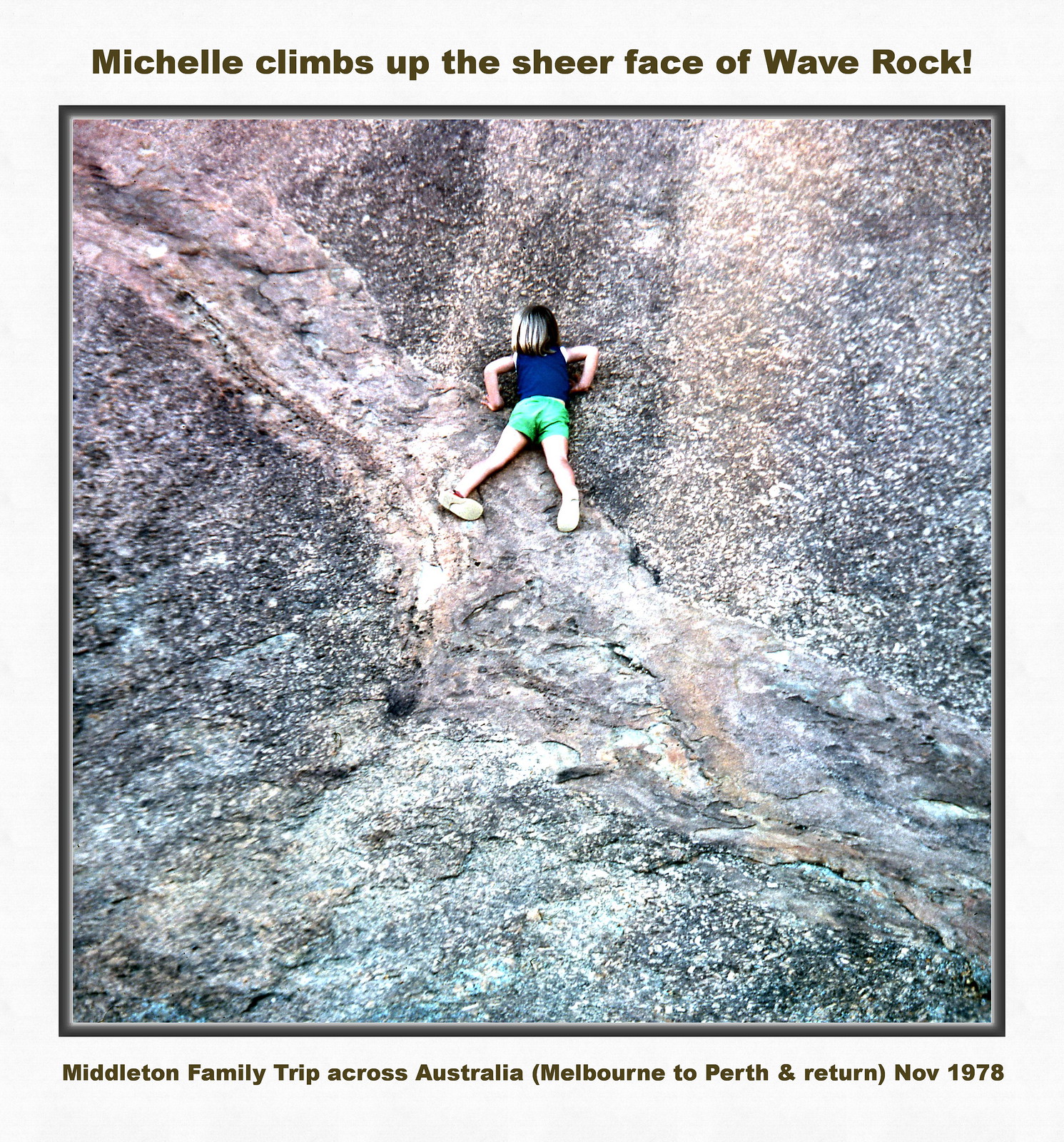This is a square-framed photograph with a grayish border, set against a whitish background, featuring an outdoor scene. The filtered image, emphasizing blue and green hues, captures a young girl climbing or possibly lying diagonally against a gray rock face with various lighter tints. She is centered slightly towards the middle-top of the frame. The child, around five or six years old, has long, shoulder-length blonde hair and is dressed in a sleeveless blue shirt, green shorts, and sneakers. The top of the image features a band of text on a light blue background stating, "Michelle climbs up the sheer face of Wave Rock!" The bottom caption reads, "Middleton family trip across Australia, Melbourne to Perth and return (November 1978)." The entire scene underscores a family adventure during their travels across Australia, highlighting a towering, stark rock face with no visible vegetation, solely varying shades of gray.